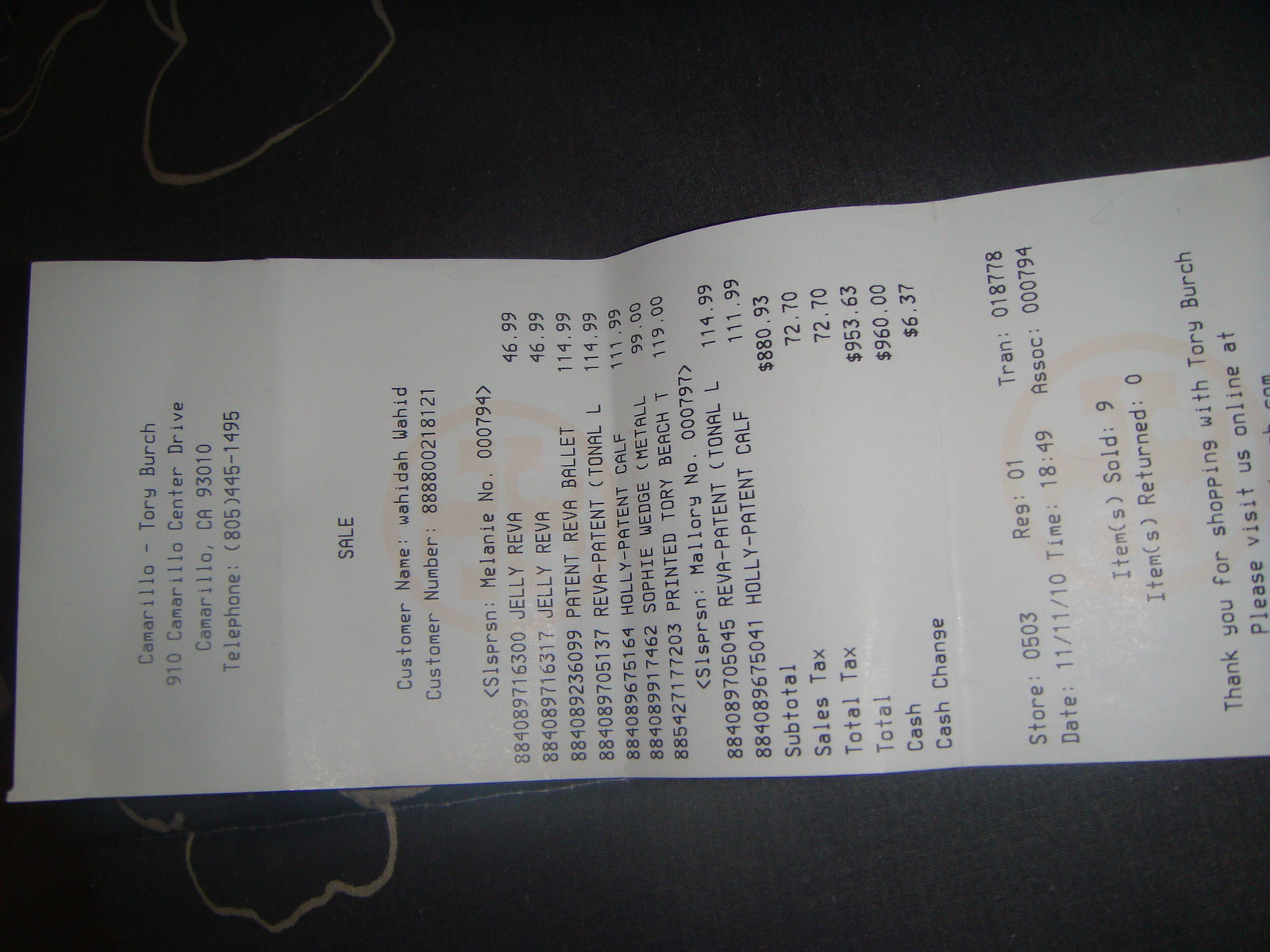This is a photograph of a receipt from Tory Burch, located at 910 Camarillo Center Drive, Camarillo, California, 93010, with the telephone number included. The receipt is printed on white paper with black text and is oriented sideways in the image. 

The receipt lists several items, including "jelly," "Patton," and various entries for "Revva Ballet," "Revva Patton," "Tonal," and "Holly Patton." The total for all items amount to $880.95, with a sales tax of $72.70, leading to a total tax-inclusive price of $953.63. The customer paid $960 in cash and received $6.37 as change.

The purchase is time-stamped at 18:49 on 11-11-2010.